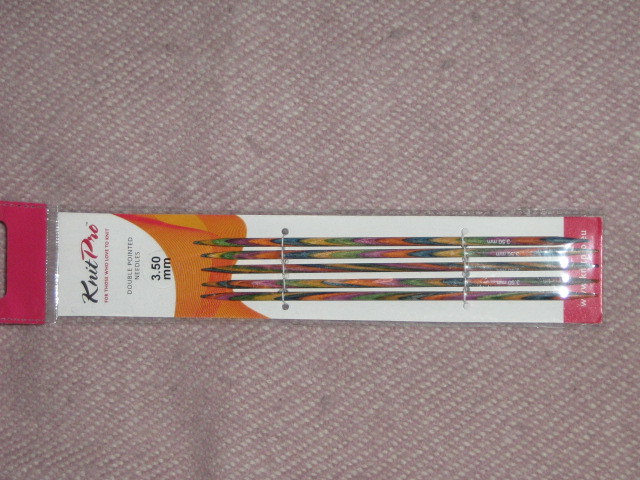This image showcases an unopened package of Knit Pro double-pointed knitting needles lying horizontally on a beige Berber carpet that has some visible dirt spots. The packaging, which is predominantly pink at the top and bottom with a white and pink design in the middle, clearly displays the brand name "Knit Pro" and specifies the needle size as 3.50 mm. The needles inside are secured with plastic zip ties and feature a vibrant, blended multicolor pattern that includes shades of pink, yellow, green, purple, orange, and red. There are five needles in total, arranged neatly within the clear package.